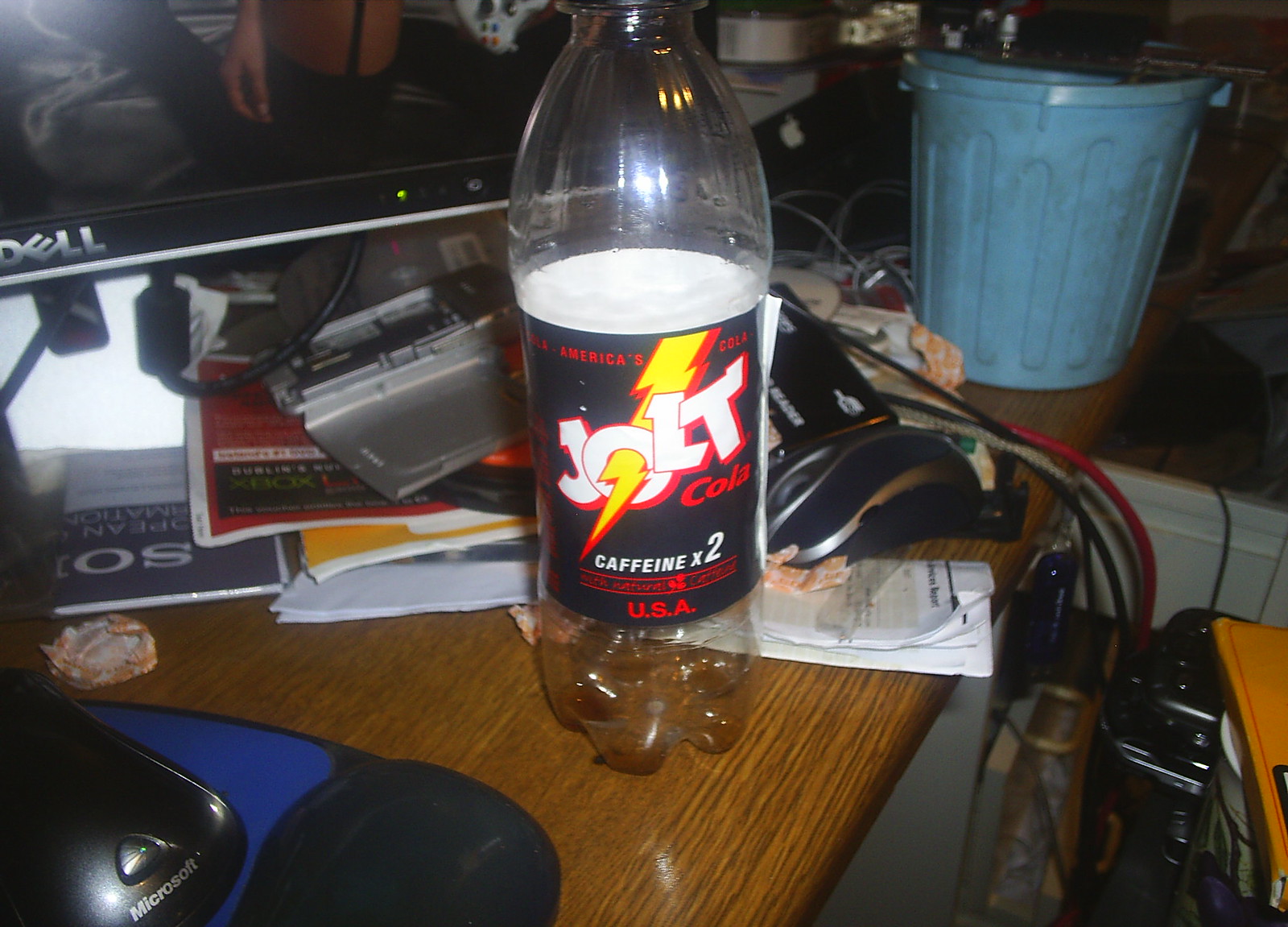An empty Jolt Cola bottle, prominently displaying the "Caffeine x2" label and "USA" branding, sits atop a cluttered wooden table. Nearby, a black Microsoft mouse rests on a mouse pad, which features a black palm rest and a blue surface. Scattered on the table is a Sony instruction manual, accompanied by a few other indistinguishable instruction booklets. A Dell-branded external monitor stands in the vicinity, along with another mouse positioned just to the right of the Jolt Cola bottle. Towards the top-right corner, a small blue trash can is visible. The scene is further complicated by a tangle of computer cables extending from the right side of the image.